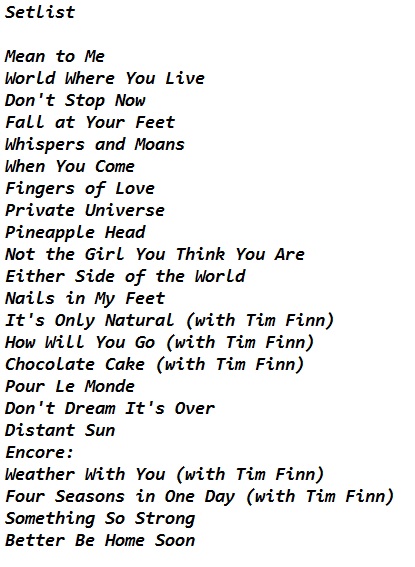The image features a stark black and white design with a basic white background covered in numerous lines of black text. Structured as a setlist, the title "Setlist" appears prominently at the top, followed by an extensive list of what appear to be song titles, each without quotation marks. The text begins with "Mean to Me," "World Where You Live," "Don't Stop Now," "Fall at Your Feet," "Whispers and Moans," "When You Come," "Fingers of Love," "Private Universe," "Pineapple Head," and "Not the Girl You Think You Are." The list continues with "Either Side of the World," "Nails in My Feet," "It's Only Natural," followed by a mention of Tim Finn collaborating on "How Will You Go," "Chocolate Cake," and "Pour Le Monde." The sequence progresses to "Don't Dream It's Over," "Distant Sun," and culminates in an "Encore" section that lists "Weather With You," again featuring Tim Finn, "Four Seasons in One Day," "Something So Strong," and "Better Be Home Soon." Remarkably, the layout is devoid of any images, icons, or banners, focusing solely on the song titles in a straightforward and unadorned presentation.